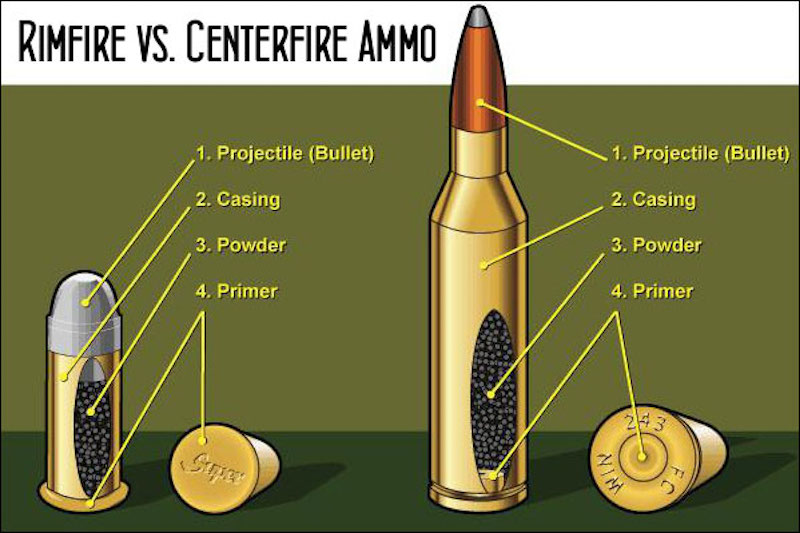The illustration, set against a light green background with a dark green surface, contrasts rimfire versus centerfire ammo. At the top left, the title "Rimfire versus Centerfire Ammo" is displayed within a white border in black letters. Below, two bullet shells are depicted: a shorter, rounded-headed silver bullet on the left, and a much taller, rifle-type bullet on the right with a copper-colored projectile and a silver tip.

Each bullet shell is sectioned to reveal its internal components, with yellow labels pointing to specific parts: "1. Projectile Bullet," "2. Casing," "3. Powder," and "4. Primer." The shorter bullet on the left has its labels pointing to the silver projectile, golden casing, visible dark powder inside, and the base primer, which is slightly wider. Similarly, the taller bullet on the right is labeled identically, emphasizing the same components but with a longer projectile and overall increased height. Both bullets are accompanied by smaller, identical bullets lying down to their right, showcasing the bottom view. The green and gold color palette helps differentiate the components clearly for comparative analysis.